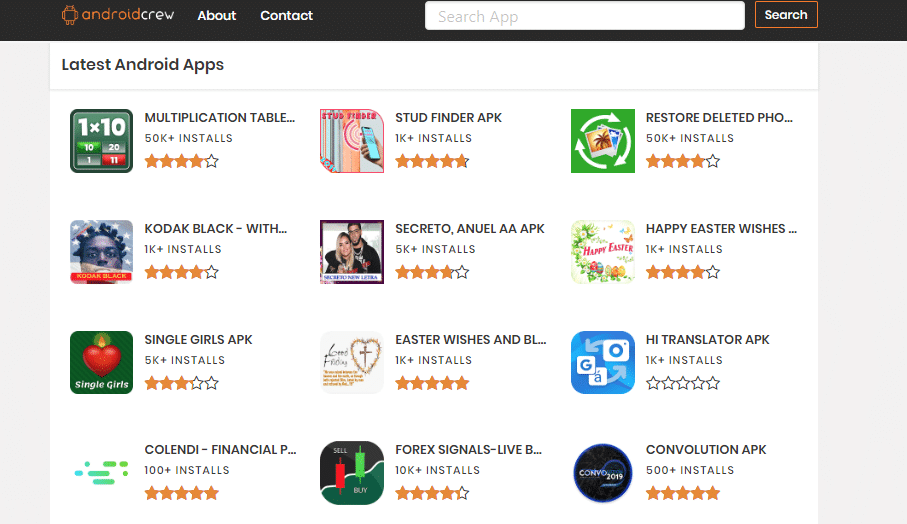**Screenshot of Android Crew Website Highlighting Latest Android Apps**

This image is a screenshot taken from a computer showcasing the user interface of the "Android Crew" website. At the top of the website, the navigation bar is visible with options such as "About" and "Contact," followed by a search box labeled "Search app." Adjacent to the search box is an orange rectangular button with black text that says "Search."

Beneath the navigation bar, in a white main content area, the heading "Latest Android Apps" is prominently displayed. Below this heading, a grid layout presents a selection of Android applications available for download, organized into four rows with three apps per row, totaling twelve apps.

- The first app in the first row is represented by a green square icon featuring the text "1x10." The app is titled "Multiplication Table" and boasts over 50,000 installs and a rating of four stars.
- Next to it, there is an app icon showing an image of a man with his arm around a woman who appears to be blonde, while the man has a darker complexion. This app is titled "Secreto, Anuel, AAPK," with over 5,000 installs and a four-star rating.

The ensuing rows continue to display various other applications, each detailed with their respective installation numbers and star ratings.